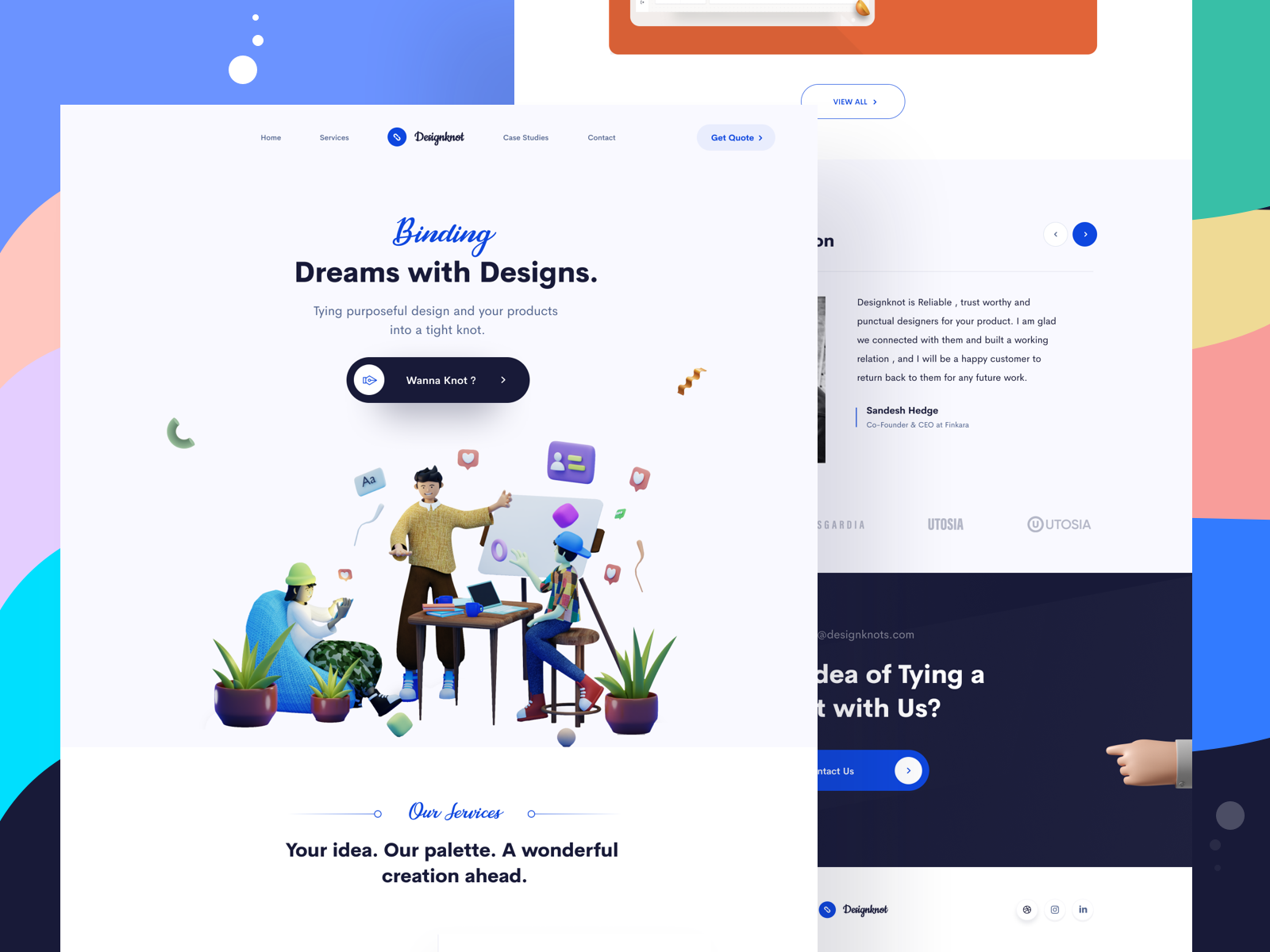The graphic showcases a layered design presentation, featuring multiple web pages merged together. The focal point is a prominent banner titled "Binding Dreams with Designs" and a tagline, "Binding purposeful design and your products into a tight knot." Below, there's a dynamic image of three 3D characters, representing artists working in a studio filled with houseplants, emphasizing creativity and collaboration. At the bottom of the main page, there's a section labeled "Our Services," which reads, "Your idea, our palette, wonderful creation ahead." The entire composition is set against a clean, white background. In the background, another page is partially visible, possibly displaying various websites that utilize the service, resembling a home page layout. In the bottom right corner, social media icons for LinkedIn and others are neatly arranged, reinforcing the connectivity and outreach of the service. The secondary page also sports a white background, maintaining a consistent and cohesive look.